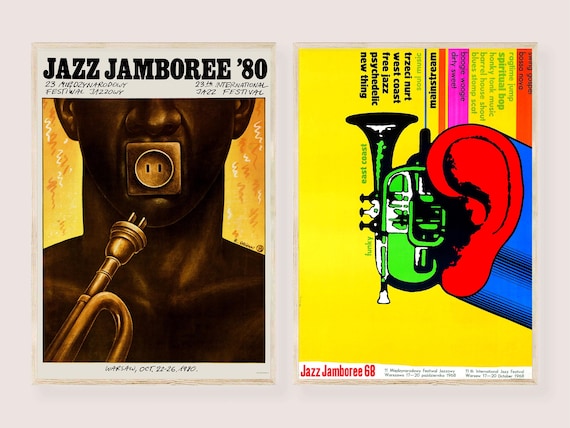This photograph showcases two side-by-side posters for the Jazz Jamboree festival, set against a white background. The poster on the left, titled "Jazz Jamboree '80," dates back to October 22-26, 1980, in Warsaw. It features the striking image of a black man with a plug receptacle in his mouth, poised to connect with an electrical plug attached to the end of his trumpet. The artwork is vibrant and intriguing, hinting at the electrifying performances of the festival.

In contrast, the right poster, labeled "Jazz Jamboree '68," presents a more cartoonish and psychedelic theme. Dominated by bold colors, the image displays a green trumpet extending from a giant red ear, with a 3D blue prismatic form emanating outward. This poster lists genres like West Coast Free Jazz Psychedelic New Thing in various colors of black and green, with much of the text oriented vertically, adding to its abstract and avant-garde aesthetic.